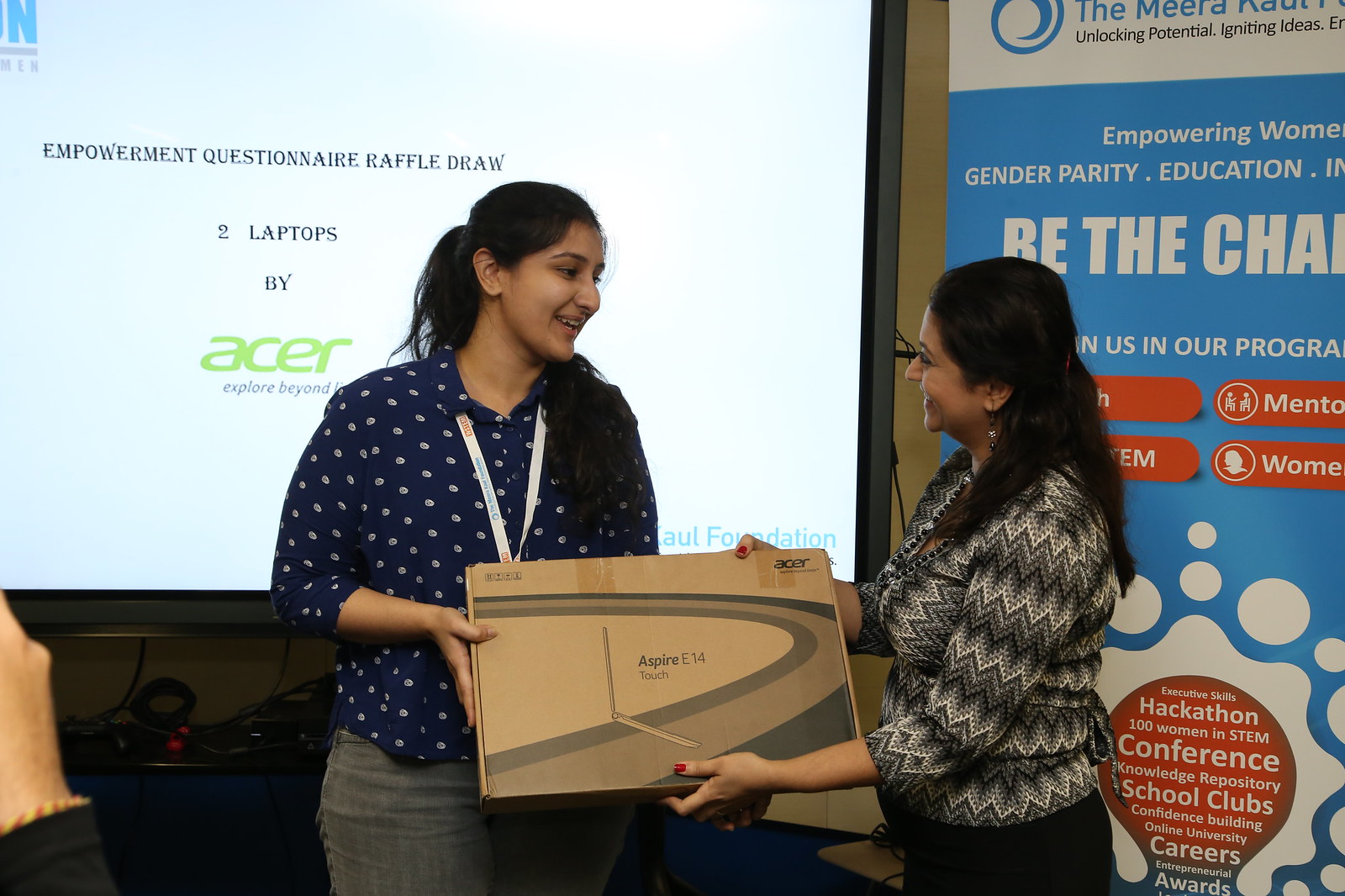In a brightly lit room, two women are central to the scene. The woman on the right, donning a zigzag-patterned black and white shirt with a black skirt, accessorized with white dangling earrings and smiling, appears to be presenting a boxed Acer Aspire E14 Touch laptop to the woman on the left. The woman receiving the box has long black hair and is dressed in a blue polka-dotted shirt with gray jeans, also smiling warmly. They face each other, sharing this moment of exchange. The background features a large screen displaying a message about an "Empowerment Questionnaire Raffle Draw" for two Acer laptops. Additionally, there is a blue cloth–covered table with some visible wires and a billboard on the far right that reads "Empowering Women, Gender Parity, Education." A hand from another person emerges from the bottom left corner, hinting at more activity in the room.